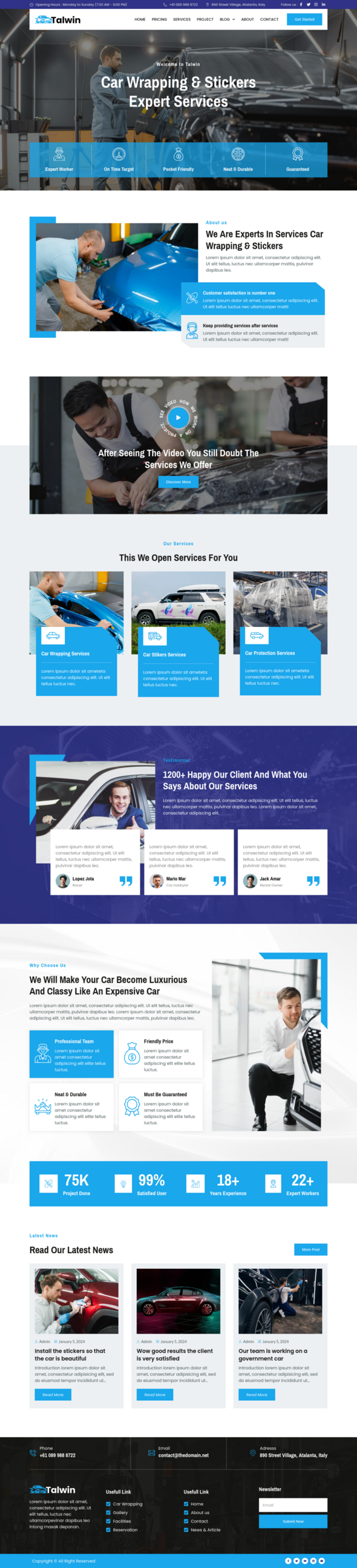This image captures the homepage of the TALWIN website. In the upper left corner, within a white navigation bar, there are seven distinct menu options listed horizontally. Adjacent to the menu is a prominent blue button. The website appears compact, making it challenging to discern finer details. Dominating the top section is a banner showcasing a scene from an auto shop where a man is actively applying wrap to a grey car. The man is oriented to the right side of the frame, situated in a garage setting that serves as the backdrop. Overlaying this image is text promoting "car wrapping and stickers, expert services." At the bottom of this banner, there's a row of five blue buttons, offering additional navigation or call-to-action elements.